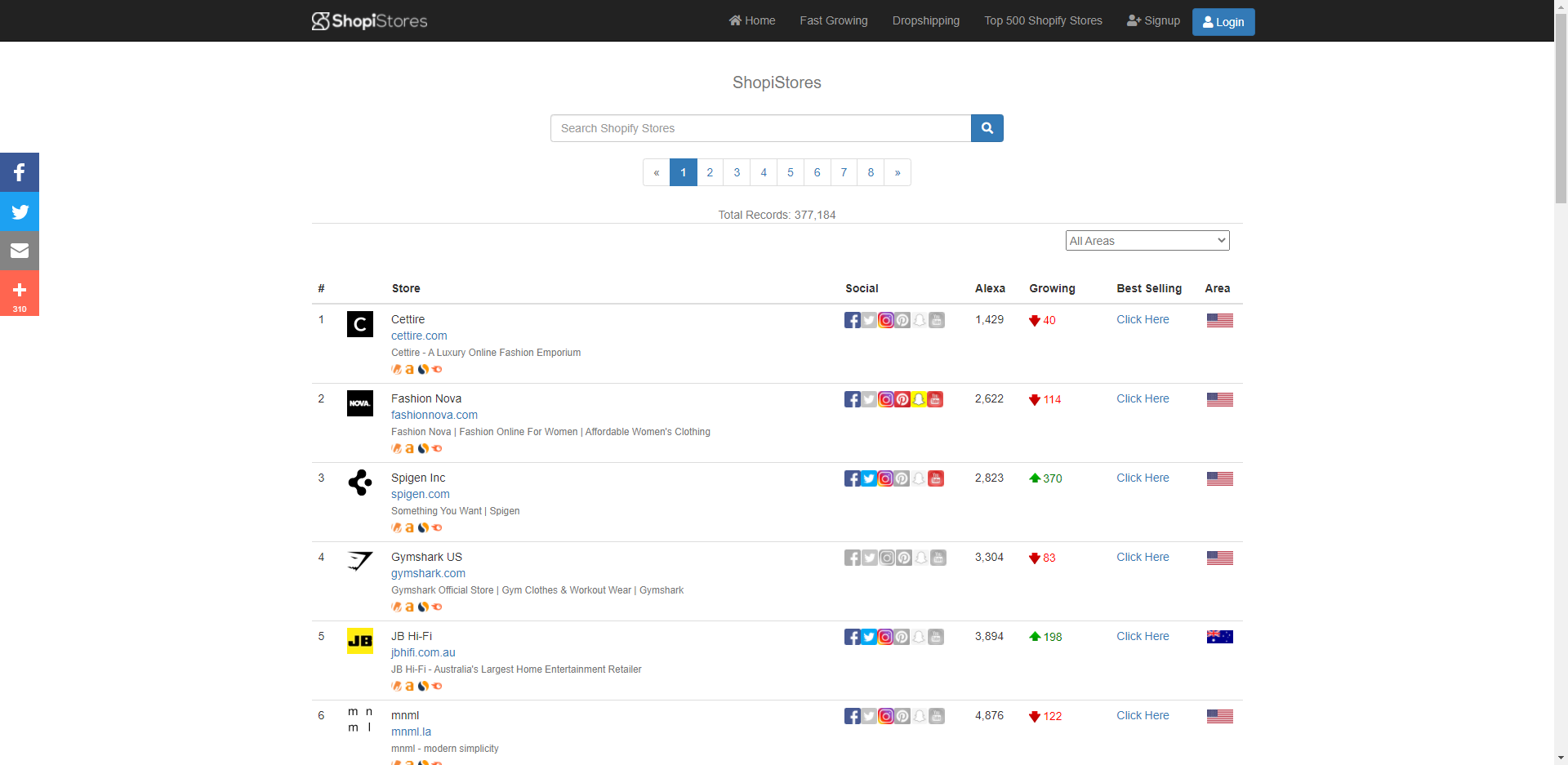In this detailed image, we observe a screenshot of a webpage dedicated to showcasing Shopify stores. In the top left corner, the heading "ShopiStores" is prominently displayed. The right side of the screen features navigation options, including "Home," "Fast Growing," "Dropshipping Top 500 Shopify Stores," "Sign Up," and "Log In." 

Centrally positioned below these functions is another large header that again reads "ShopiStores," followed by a search bar with the placeholder text "Search Shopify Stores." The main section of the page displays a grid of eight small squares, arranged in two rows of four, accompanied by the label "Total Records: 377,184." On the far right of this grid, a dropdown menu labeled "All Areas" is visible.

Below the grid, a list enumerates the top six stores:
1. Satire
2. Fashion Nova
3. Spicken Incorporation
4. Gymshark US
5. JB Hi-Fi
6. MNML

Additionally, on the right-hand side of the screen, there is a social tab featuring categories such as "Alexa," "Growing," "Best-Selling," and "Area," likely intended for further filtering or information about the stores.